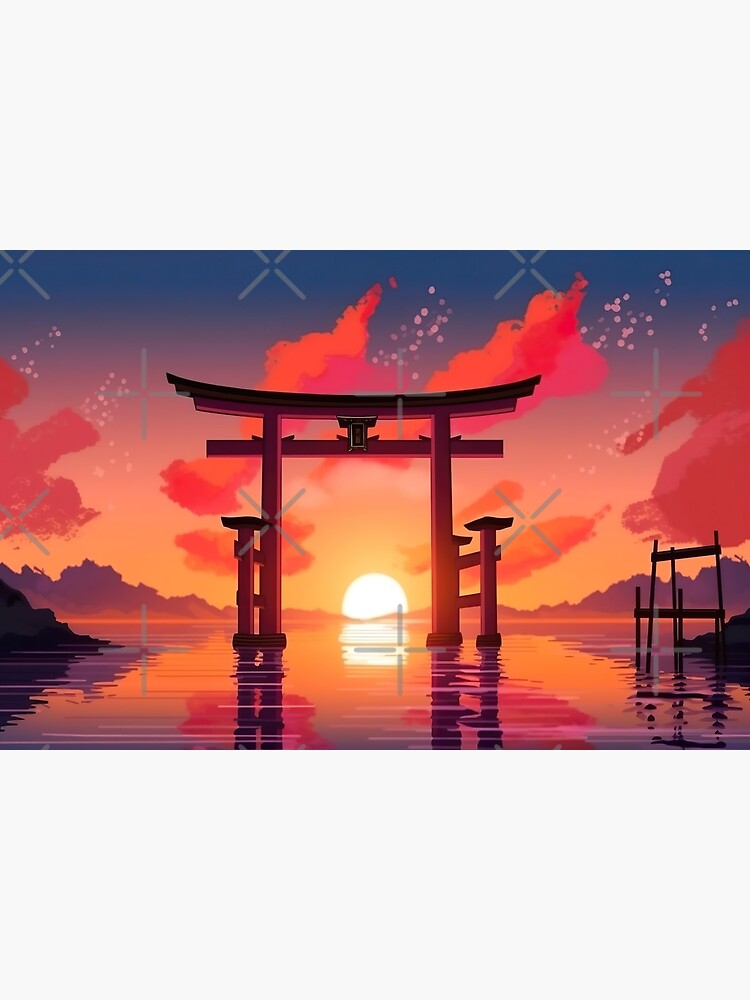This digital illustration depicts a serene sunset over a body of water, dominated by a striking red torii gate at its center. The torii gate, an iconic structure in Japanese culture characterized by its arches and horizontal beams, rises majestically from the water, appearing almost symmetrical on both sides with a slightly concave top. The sky above transitions from a deep blue at the top to a warm gradient of purples, pinks, and oranges closer to the horizon, where the almost fully set, brilliant yellow sun casts its golden reflections on the rippling water below. Flanking the scene are silhouettes of distant mountains, their shapes subtly mirrored in the tranquil waters. Wispy clouds, streaked in hues of orange, red, and pink, drift across the sky, while faint outlines of stars begin to appear. The overall color palette beautifully captures the essence of a peaceful evening, blending blues, yellows, pinks, and purples to enhance the tranquil ambiance of this Asian-inspired setting.